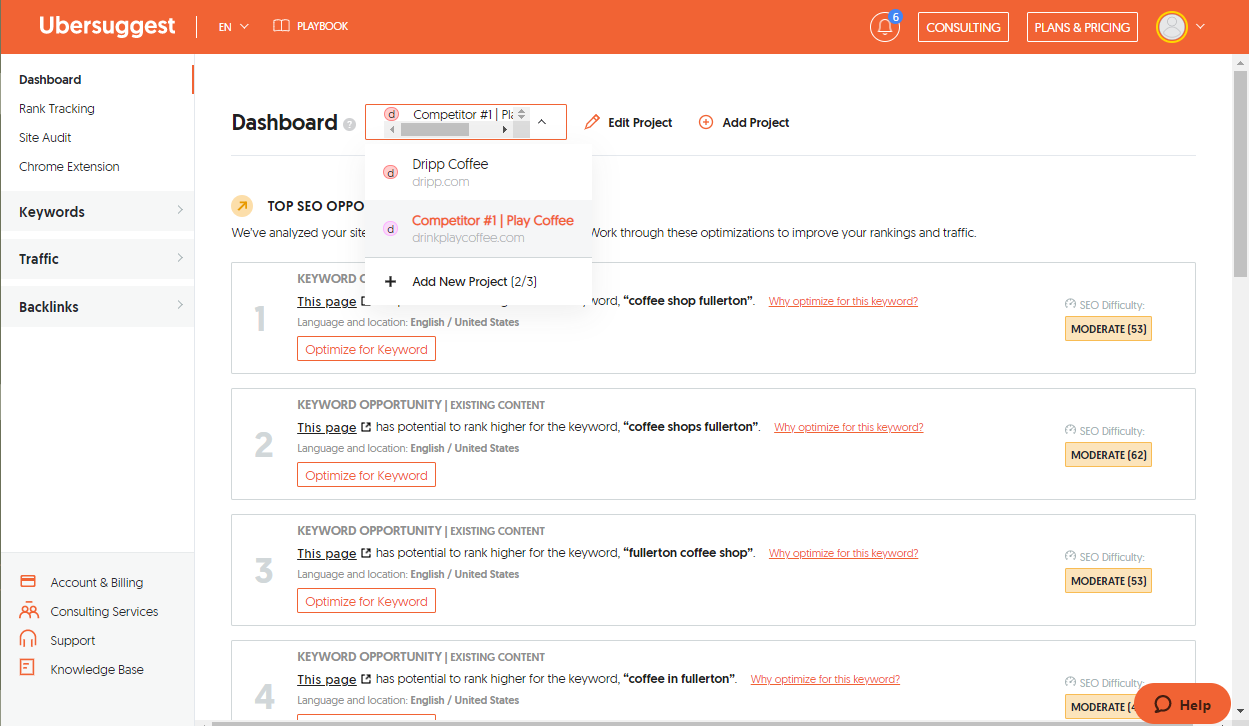**Detailed Caption:**

This is a detailed screenshot of a web page from Ubersuggest. The header of the webpage is prominently highlighted with an orange bar that includes several elements. On the upper left hand side of the orange bar, "Ubersuggest" is displayed in white, capitalized text. Directly next to this is a vertical bar, followed by a language selection option showing "EN" with a downward arrow indicating a dropdown menu. Adjacent to this, there is an icon of an open book labeled "Playbook". Towards the right end of this orange header bar, there is a bell icon encircled, which has a smaller blue circle in its upper right corner displaying the number six in white text. Flanking these are two buttons labeled ”Consulting” and “Plans and Pricing”. Concluding this segment on the far right is a circular icon with a yellow outline and a bluish-green center, featuring a person icon with a downward arrow for a dropdown menu.

Below the header, the main body of the website is organized into a dashboard layout. On the leftmost section, there are various navigation options. The primary menu items include "Dashboard" in bold black text, followed by options such as "Rank Tracking,” "Site Audit," and "Chrome Extension." These are each displayed in regular black text. More menu options like "Keywords," "Traffic," and "Backlinks" are highlighted in bold black text on a light gray background. Further down this left sidebar, additional options like "Account and Billing," "Consulting Service Support," and "Knowledge Base" can be found.

In the central dashboard area, the page contains several key functionalities. On the upper left corner, you can find options like "Edit Project" and "Add Project." Below this, a section reveals top SEO results, clearly itemized and numbered from 1 to 4. Each entry features a description of the results, with a button labeled "Optimize Keyword" for each of the four options. The numbers are displayed in light gray text with a gray outline.

On the rightmost part of the dashboard, there is a slider bar, and in the lower right corner, a "Help" button is featured. This button is represented by a black quote bubble with the word "Help" written in black text on an orange background.